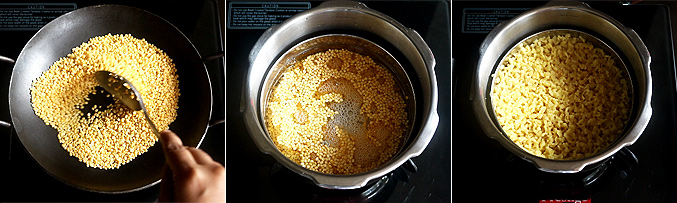This is a detailed, step-by-step time-lapse of cooking pasta in a black wok and then finishing the process in a pressure cooker-like pot. In the first image on the left, you can see a hand stirring small, dry twirly-shaped pasta with a large metal spoon that has holes in it. The pasta is placed in a black wok with a metal rim. In the second center image, the pasta is submerged in water inside a large silver pot resembling a pressure cooker or steamer. The water is boiling, and you can see bubbles indicating active cooking on a black stovetop burner. In the final image on the right, the now-cooked pasta has expanded and is sitting in the strainer inside the larger pot. The transformation from small, dry pasta to large, cooked pieces is clearly visible across the three images.